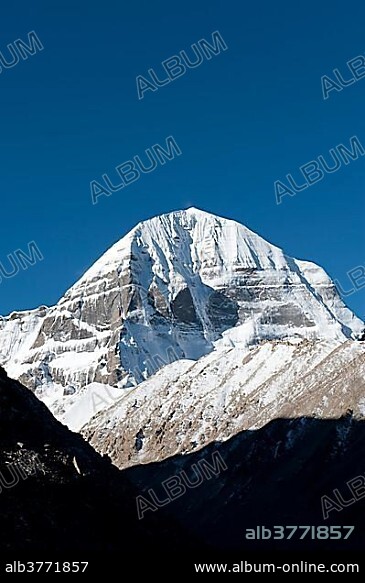This image, featured on the webpage www.albumonline.com, showcases a tall, blunt, and rocky mountain adorned with patches of snow, indicating its high-altitude location. The sheer, rocky sides of the mountain are distinct, with snow visibly collected at the base and scattered across various spots. The base descends into a dark, silhouetted valley marked by signs of rock slides and fallen rock chunks. The sky in the upper half of the image is a deep, bright blue, providing a stark contrast to the snow-covered peak and the shadowed valley below.

This stock photo is marked with several identifiers: the number ALB3771857 appears in the lower left corner in white letters, and once more in blue letters slightly above it. The URL www.album-online.com is displayed in white letters in the lower right corner. Additionally, the word "album" is watermarked in blue bubble letters across the image, slightly tilted so that the 'A' is positioned below the 'M.'